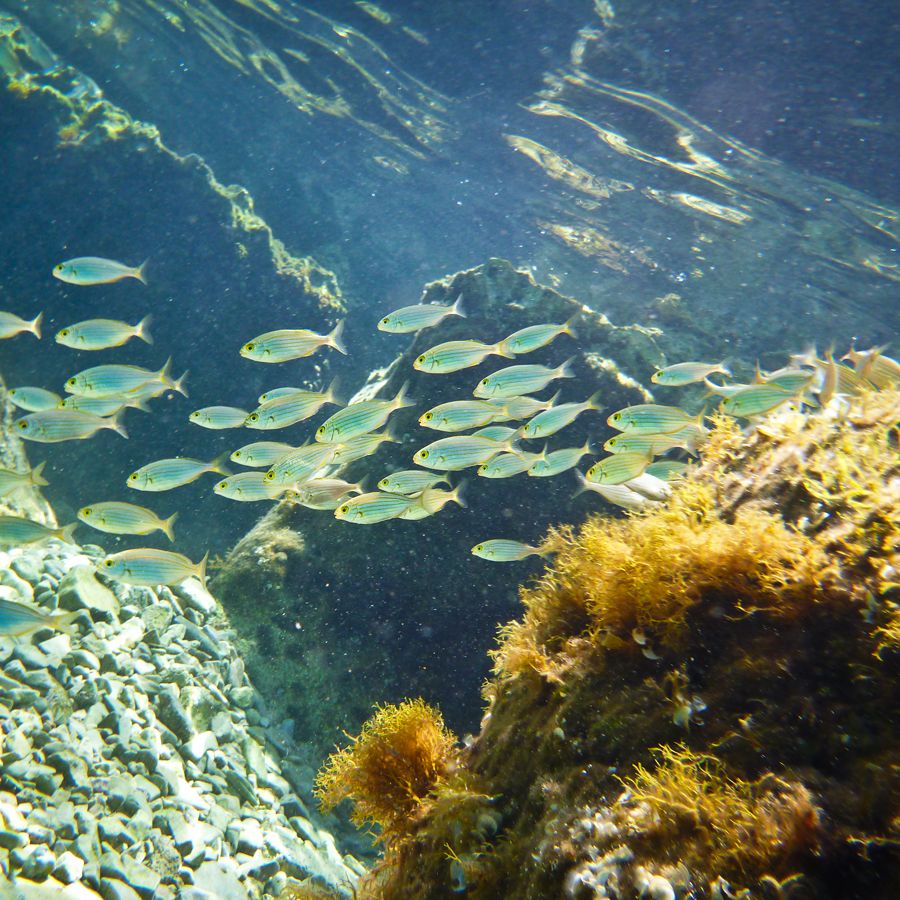This underwater scene captures a vibrant and bustling coral reef environment. Dominating the image is a school of medium-sized fish, their bodies exhibiting a bluish-green hue with silvery undertones and striped designs. These fish are swimming collectively towards the left side of the frame, blending harmoniously with the background due to their coloration. The bottom right corner showcases a cluster of orange and yellow coral or sea plants, enlivening the rocky substrate they grow upon. Contrasting this, the bottom left corner is strewn with gray and white rocks and pebbles, adding texture to the scene. Majestic rock formations rise in the background, creating a dramatic underwater landscape. Near the top, the water's surface is visible, with sunlight piercing through, generating ripples and white highlights that dance across the scene. The image beautifully encapsulates the intricate and lively ecosystem of the ocean's depths.